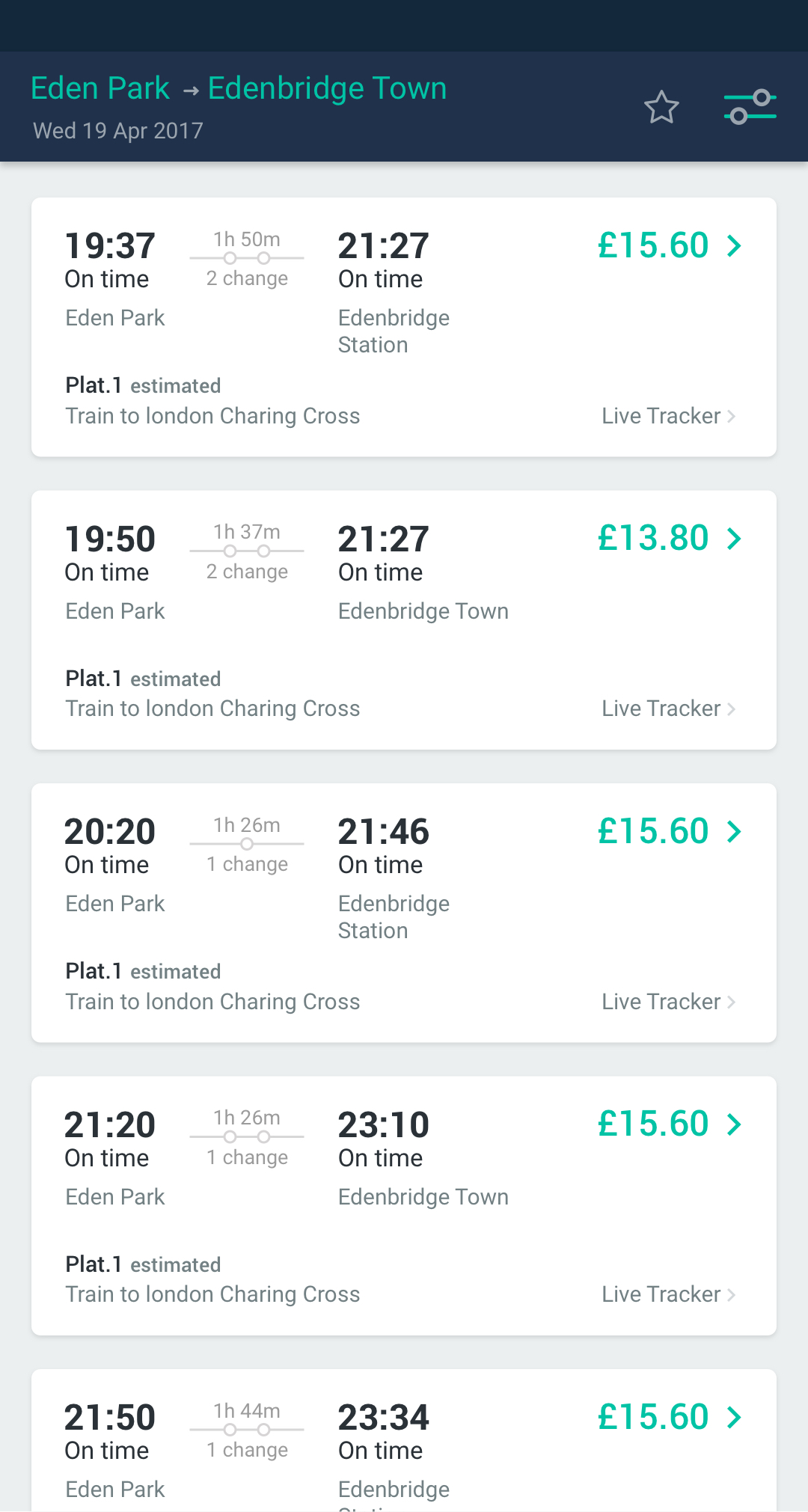Screenshot of a mobile application displaying various train schedules from Eden Park to Edenbridge Town on Wednesday, 19th April 2017. The app interface is styled with a navy blue border at the top. Within this border, in green font, the route and date are highlighted: "Eden Park to Edenbridge Town, Wednesday, 19th April 2017." To the right, there's a grey star icon next to a grey and green filter icon. 

Detailed schedules and fares are listed as follows:
- The first entry shows a departure at 19:37 from Eden Park, with an estimated arrival at 21:27 at Edenbridge Town, requiring a 1-hour 50-minute change. The train is expected to arrive at Platform 1 at London Charing Cross, with a fare of £15.60.
- The second entry indicates a 19:50 departure from Eden Park, arriving at 21:27 at Edenbridge Town after a 1-hour 37-minute change. This service also heads to London Charing Cross, costing £13.80.
- The third entry lists a 20:20 departure from Eden Park, arriving at 21:46 at Edenbridge Town with a 1-hour 26-minute change, with one change required and a fare of £15.60.
- The fourth entry shows a 21:20 departure from Eden Park, arriving at 23:10 at Edenbridge Town. This journey takes 1 hour 26 minutes, requires one change at Platform 1, and costs £15.60.
- The last entry details a 21:50 departure from Eden Park, arriving at 23:34 at Edenbridge Town after a 1-hour 44-minute journey with one change, priced at £15.60.